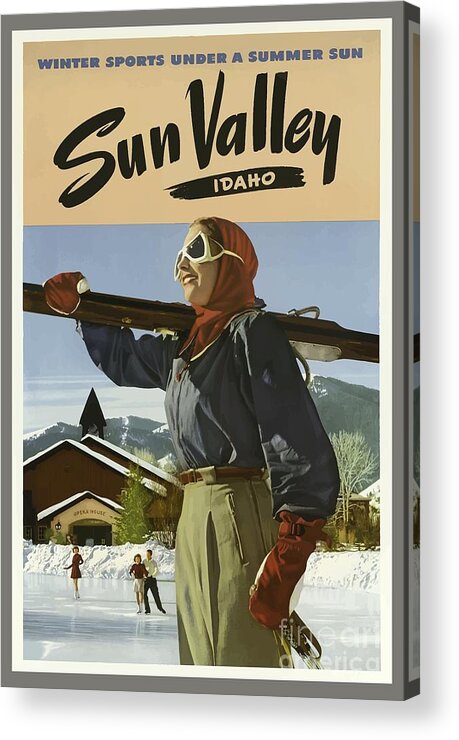This is a color image of a vintage-style poster promoting Sun Valley, Idaho, resembling those created during the Great Depression to advertise American leisure destinations. The poster, likely displayed in train stations or airports, measures approximately four feet tall by three feet wide. At the top, a tan horizontal stripe features the slogan, "Winter Sports Under a Summer Sun," in gray letters, followed by "Sun Valley" in black and "Idaho" in tan letters on a black stripe below. The central figure is a woman clad in vintage ski attire: a red scarf wrapped around her head and neck, white-framed snow goggles, and a dark blue long-sleeved blouse. She is holding a pair of skis over her right shoulder and carries snow poles in one hand, while sporting red mittens and olive-colored, khaki-style slacks. Her belt is brown, and she is depicted against a backdrop of a snow-covered skating rink with three skaters—two women and one man—gliding on the ice. Beyond the rink, a church with a steeple is visible to the left of the woman, set against snow-capped mountains beneath a partly cloudy blue sky.